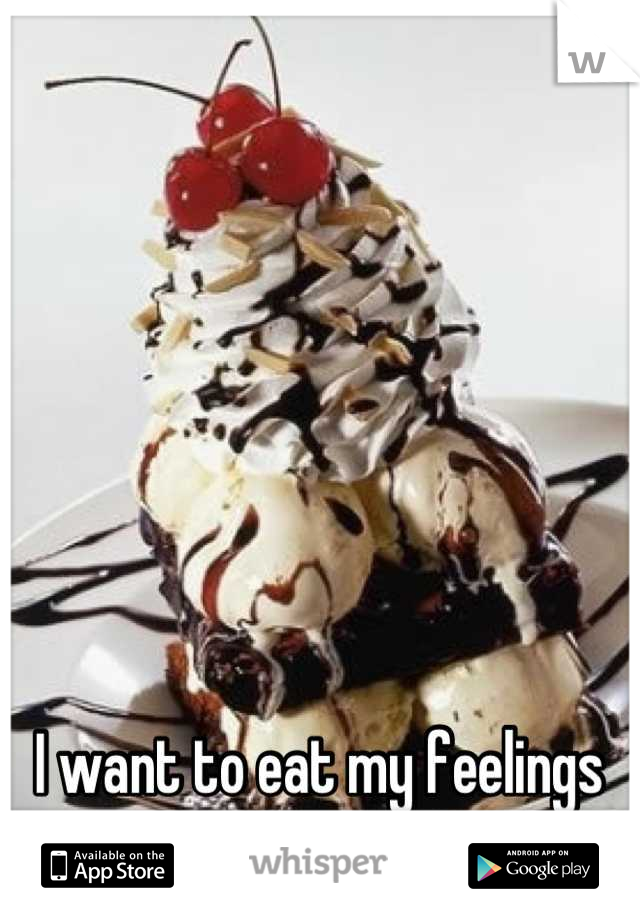The image is a detailed close-up of a decadent ice cream sundae positioned diagonally in the center of the frame against a white background. This sundae features several layers starting with a base of rich brownies, followed by scoops of vanilla ice cream, and is topped with generous swirls of whipped cream. Adorning the sundae are various toppings including a drizzle of chocolate syrup, crunchy nuts, and cherries, with a striking chocolate wafer adding height. The white plate underneath also bears a splash of chocolate sauce. The arrangement of the sundae, resembling a slightly leaning cone, is visually striking, showcasing colors of red, white, yellow, black, and brown. In the upper right corner of the image, there's a logo—a triangle with a 'W' inside. At the bottom, against a strip of pure white, text reads "I want to eat my feelings." Flanking this central text are black rectangles indicating availability on the App Store and Google Play, with the word "Whisper" in gray text in between, identifying the image as an ad for the Whisper app.